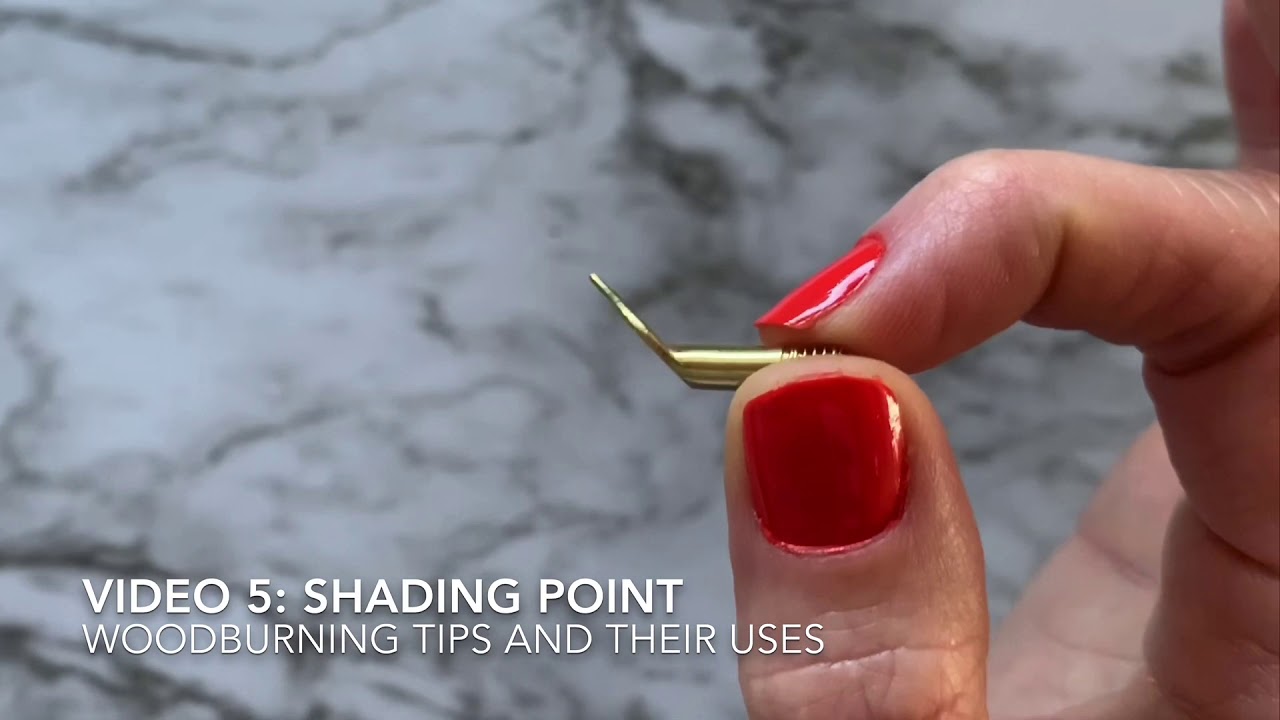This image, resembling a still from a video, features a close-up of a hand with bright reddish-orange nail polish, albeit messily applied around the cuticles, holding a brass-colored, screw-threaded wood-burning tip. The object, described as having a flat plate extending at an odd angle from its cylindrical form, is pinched between the index finger and thumb. Superimposed on the image is white text that reads, "Video 5: Shading Point, Wood Burning Tips and Their Uses." The background displays a black and white marble surface, possibly a counter or a table, adding contrast to the detailed presentation of the wood-burning tool.